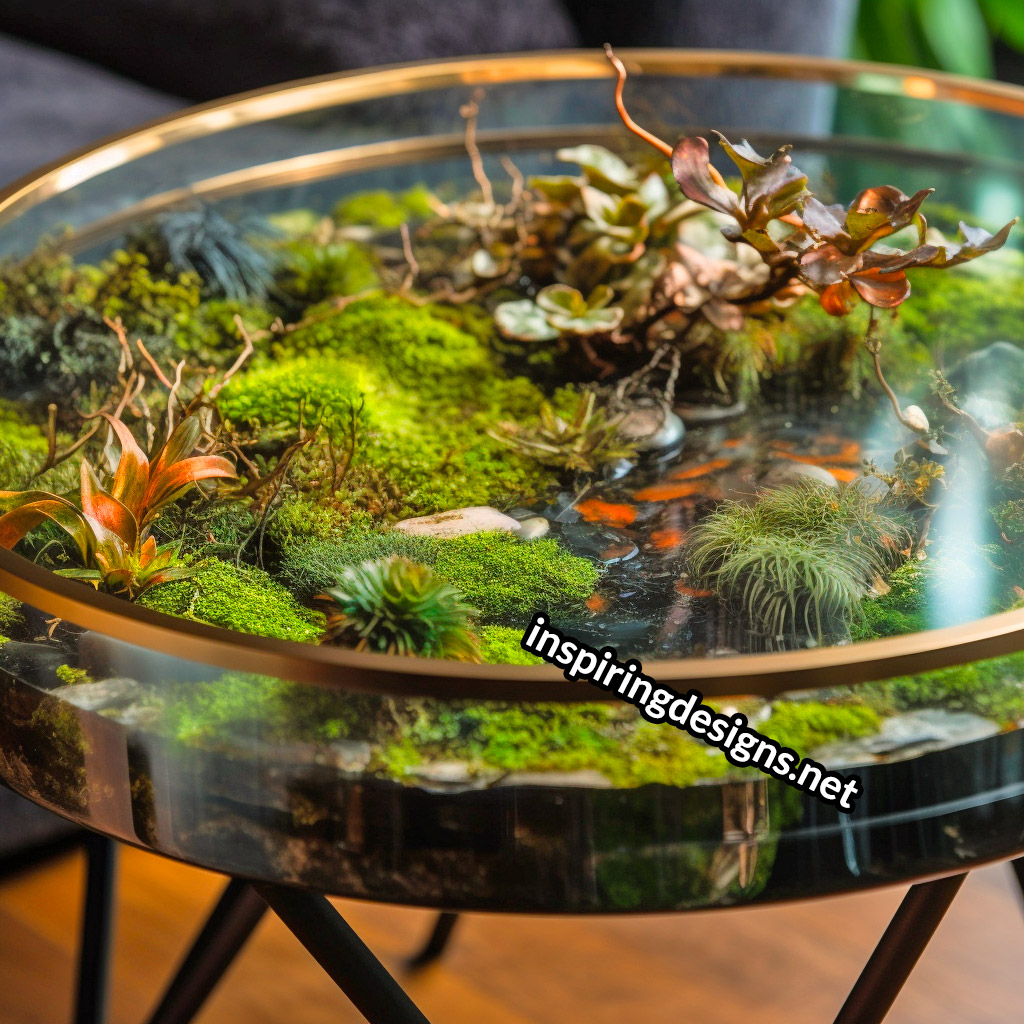The photograph captures a unique and artistic table adorned with a meticulously crafted miniature wetland environment. The table is topped with a glass enclosure framed by a gold rim, under which black metal triangular shapes act as supportive feet. The centerpiece boasts a variety of mosses and lush green plants imitating a natural wetland setting, complete with a central pond area populated by miniature goldfish. The blurred backdrop hints at a dark gray and green room, possibly including a gray couch, and the table itself appears to be set on a wooden or partially marble surface. An overlay text watermark reading "inspiringdesigns.net" is prominently displayed in white font on a black background, indicating the source of this inspiring interior design piece.